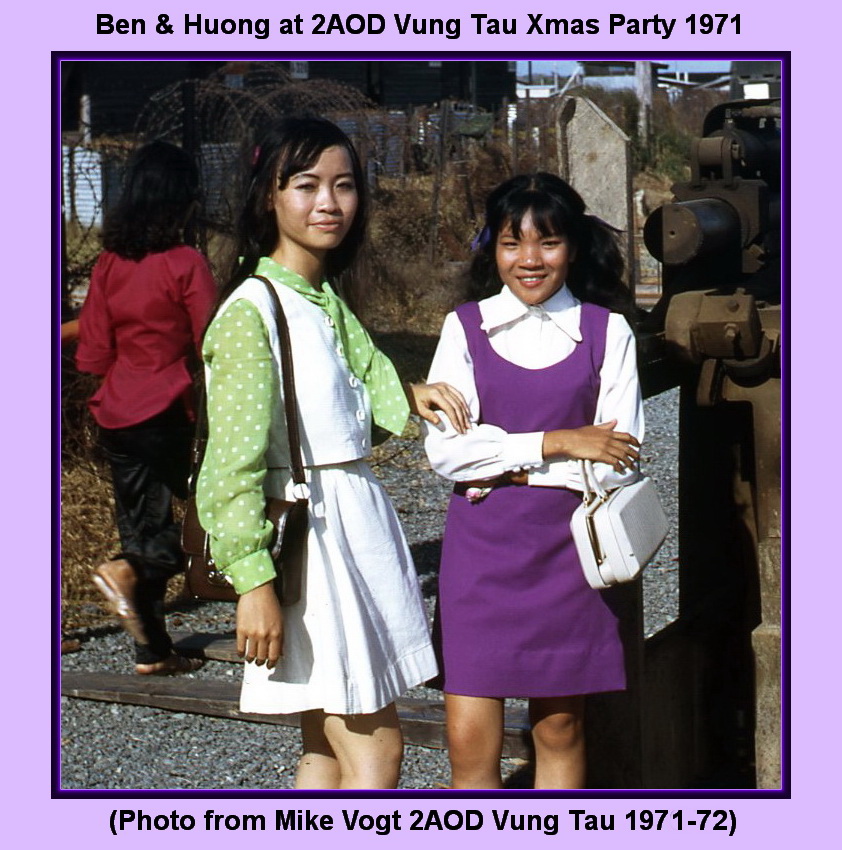This image features two Vietnamese women at the 2AOD Vung Tau Christmas Party in 1971, a scene from the Vietnam War era. At the top of the postcard-like border reads "Ben and Hoang at 2AOD Vung Tau Xmas Party 1971," while the bottom notes "Photo from Mike Vogt, 2AOD Vung Tau 1971-72." Both women, likely in their early adulthood, stand prominently in the center against an outdoor backdrop. The woman on the left is dressed in a white dress with a medium green collar and sleeves, positioned slightly to her side but glancing back towards the camera. The woman on the right wears a purple and white dress, facing directly forward with a smile. Both have medium length dark hair. In the background, to the left, a person in black pants and a silver white long-sleeved shirt walks away from the camera. The scene includes rusty metal equipment and brushes, mostly in shades of white, green, purple, red, and brown. A stone walkway is visible, adding to the rustic outdoor setting.